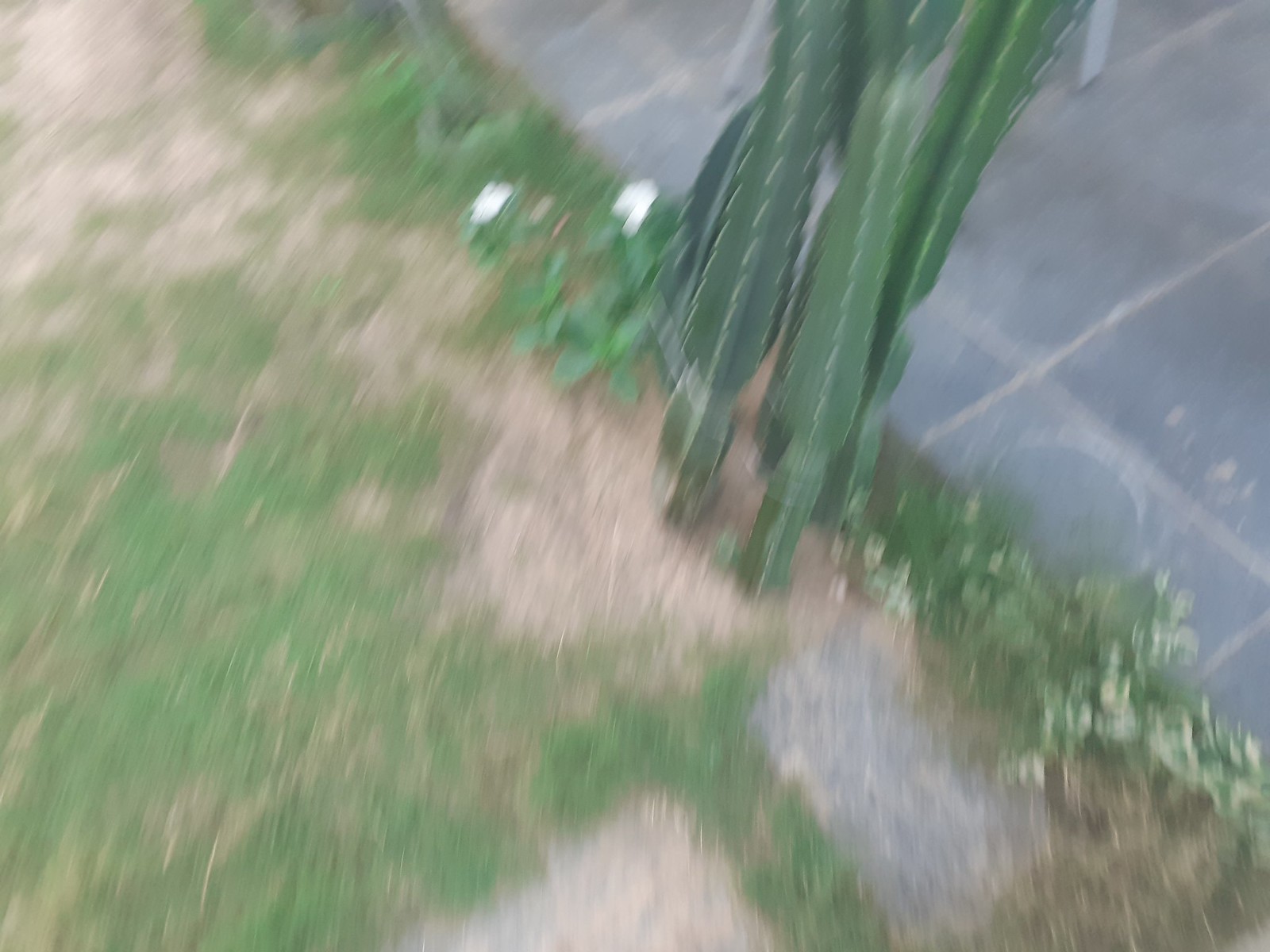This slightly out-of-focus photograph captures a ground-level scene featuring a patchy grass area interspersed with dirt and small tufts of grass. The grass patches extend up to the edge of a grey-tiled walkway or patio, which is delineated by light grey mortar. The tiles appear to be of a slate variety, laid in a neat, structured arrangement. Nestled along the border where the grass meets the tiled path, a cluster of delicate white flowers can be seen, providing a gentle contrast to the surrounding greenery. Adjacent to these flowers, a sharp, tall green cactus stands out prominently. Additionally, the leg of a chair intrudes into the frame, hinting at nearby seating and adding a subtle human element to the scene.